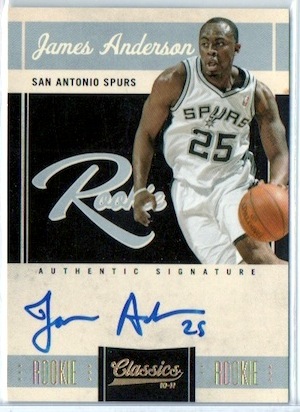The image features a basketball player wearing a white San Antonio Spurs uniform adorned with black lettering. The tank top bears the word "SPURS" in capital letters across the chest, along with the number "25" prominently displayed. He is dribbling a basketball with his left hand and looking to the left. The background consists of a large black block, with the word "rookie" inscribed in gray text. Above the player, a grayish-blue banner contains cursive text that reads "James Anderson," followed by another section in black text indicating "San Antonio Spurs." Below the player's image, a beige banner features his signature in blue marker next to the number "25," labeled with "authentic signature" in black text. The player's white shorts complement his tank top, both outlined and striped with black, emphasizing his status as a rookie from the 2010-2011 season.